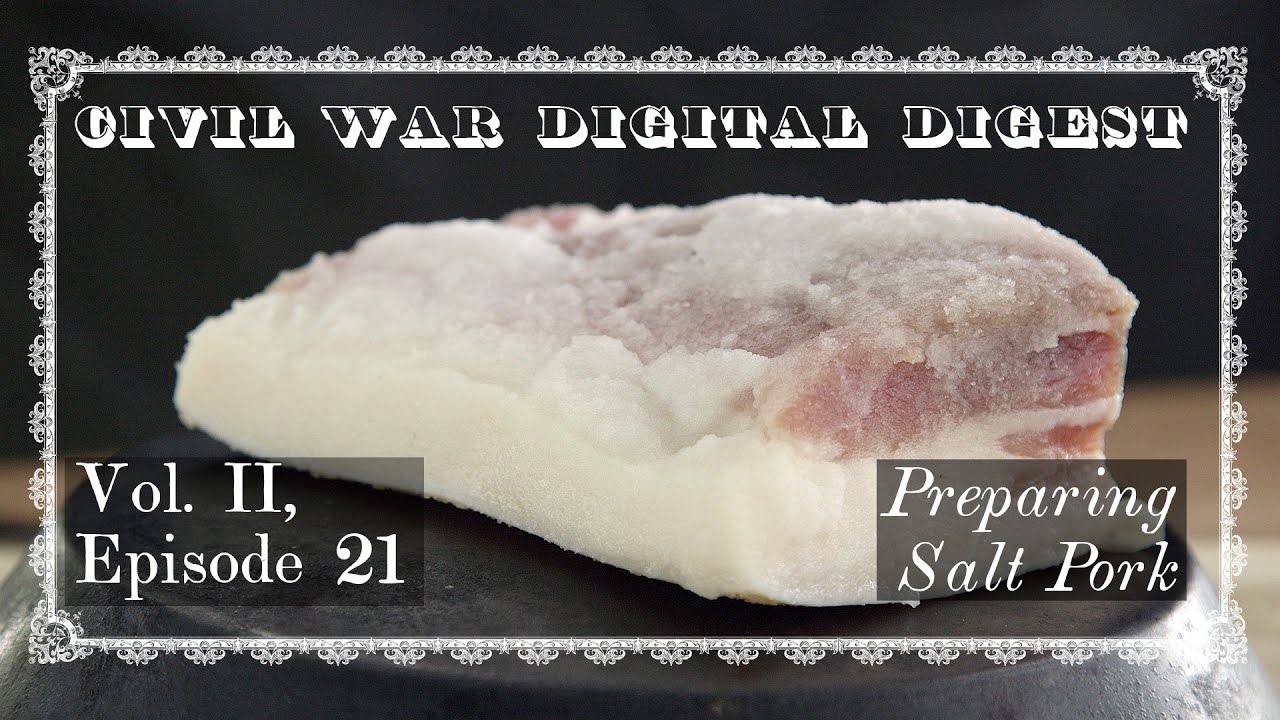This is a black-and-white image framed by an intricate white border with crown-like designs. Dominating the center is a piece of salt pork, colored dark red and interspersed with white from the fat. The pork is taller on the right side and appears sprinkled with salt or another substance. At the top of the image, black text with a white shadow reads "Civil War Digital Digest." In the bottom left corner, it says "Volume 2, Episode 21," and in the bottom right corner, "Preparing Salt Pork." The content hints at an introduction to a historical video series on Civil War-era cooking methods.